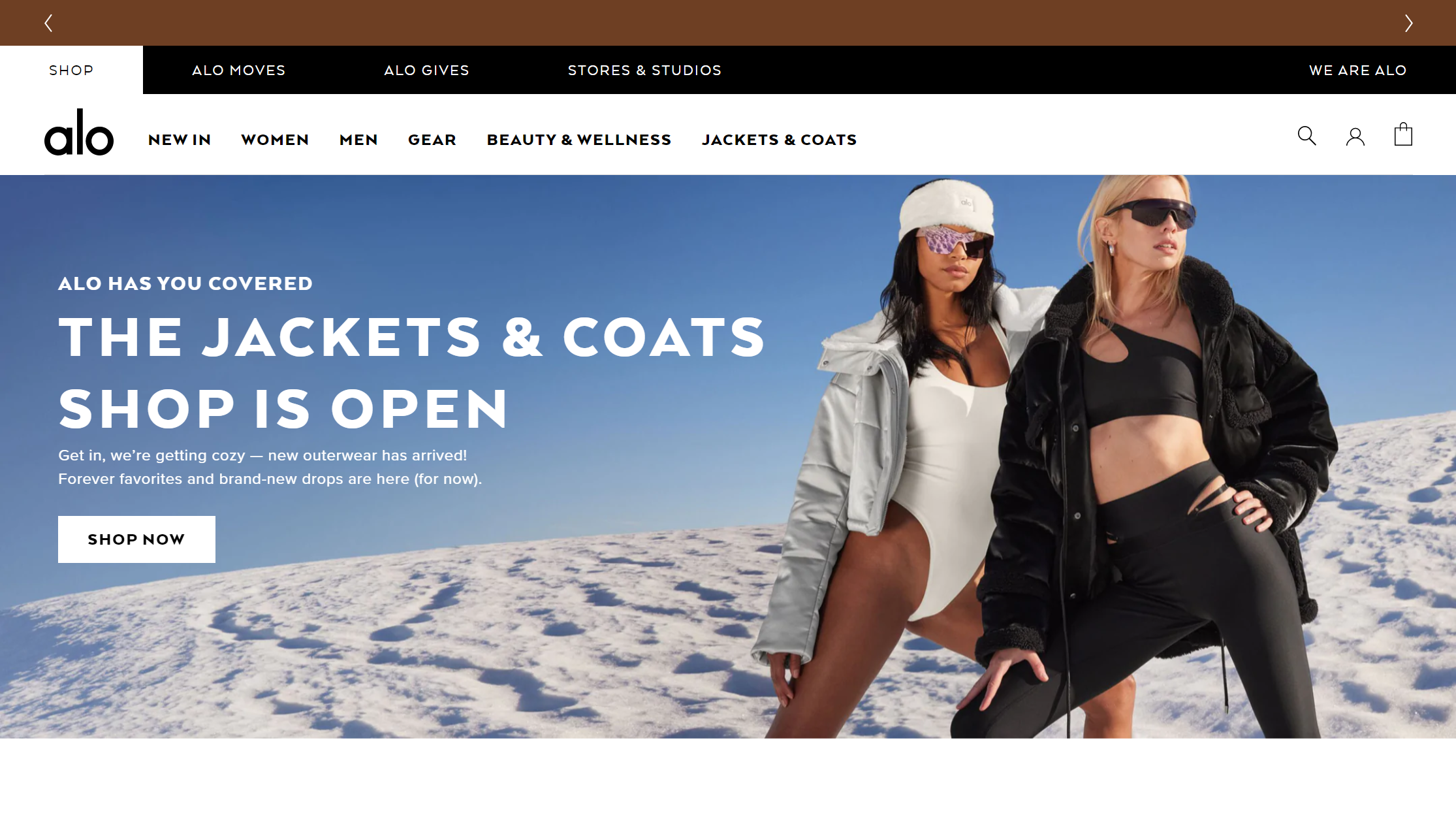The image showcases the homepage of the new fashion site, Allo (A-L-O). At the very top of the page, there is a brown banner followed by a white band that features the word "Shop." Below this is a black section with headings such as "Allo Moves," "Allo Gives," and "We Are Allo." Further down, another white band displays additional menus including "New In," "Women," "Men," "Gear," "Beauty and Wellness," and "Jackets and Coats."

The main feature of the website is a striking image of a snowscape with a vivid blue sky. In the center of the snowy landscape stand two women dressed in bold, contrasting outfits presumably available from Allo. One woman is clad in a white leotard paired with a white jacket, while the other sports a black leotard and black jacket. The unexpected choice of attire in a snowy setting captures attention immediately.

Overlaying the bright blue sky is text that reads, "Allo has you covered. The jackets and coats shop is open. Get in, we're getting cozy. New outerwear has arrived." Below this inviting message, there is a "Shop Now" button encouraging visitors to explore the new collection.